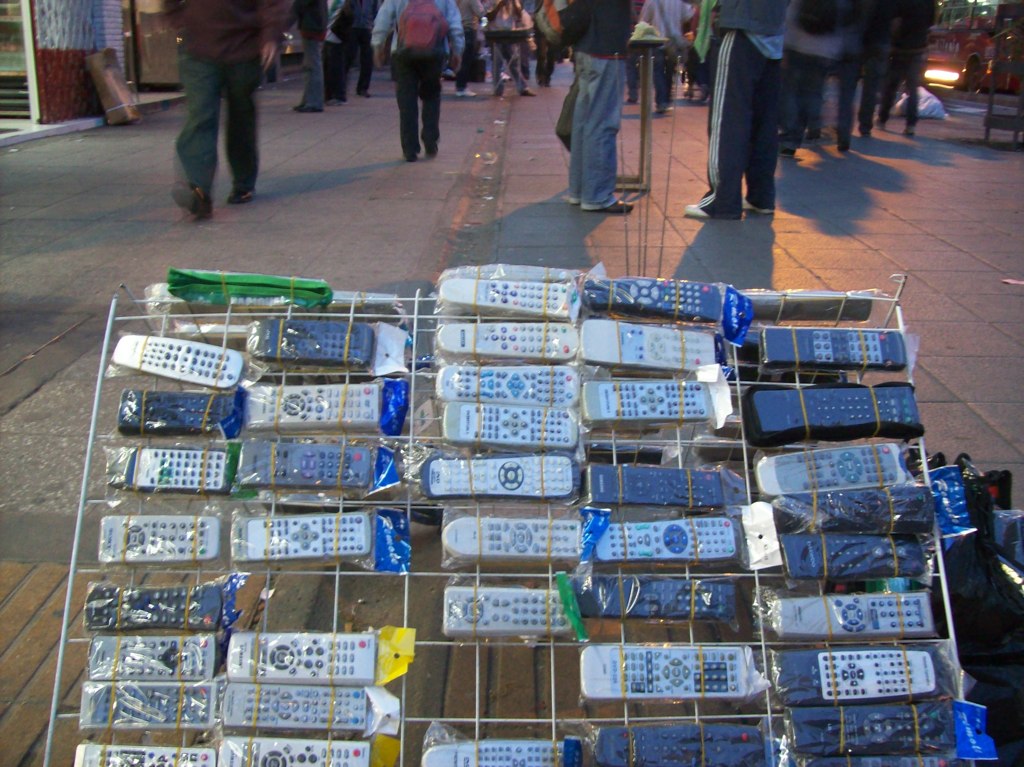This detailed image captures a street vendor's setup showcasing numerous universal TV remotes. These remotes are encased in plastic packaging and secured with golden rubber bands to a white, V-shaped wire rack. The rack itself is made of a thin metal painted white and tapers towards the back, presumably holding remotes on both sides. 

The remotes come in various colors, primarily black, silver, and white, with some featuring green, blue, or yellow accents and buttons of differing colors, including light grey, red, and blue. In total, there appear to be around 40 remotes visible on this side of the display.

Situated on an outdoor pavement, which consists of a mix of grey tiles and yellow bricks, the scene is set during daylight, possibly at sundown. In the background, a number of people are milling about, although the photograph cuts off at their waists, leaving only their lower halves visible. These pedestrians are dressed casually in jeans, tracksuits, t-shirts, shorts, and sneakers, and some carry backpacks. The pavement also features a brickwork inlay extending towards the display, and there are glimpses of building entrances or booths nearby, hinting at a possible marketplace setting.

Overall, the focus remains sharply on the array of universal remotes in the foreground, highlighting the details of their arrangement and the bustling street environment in which they are being sold.